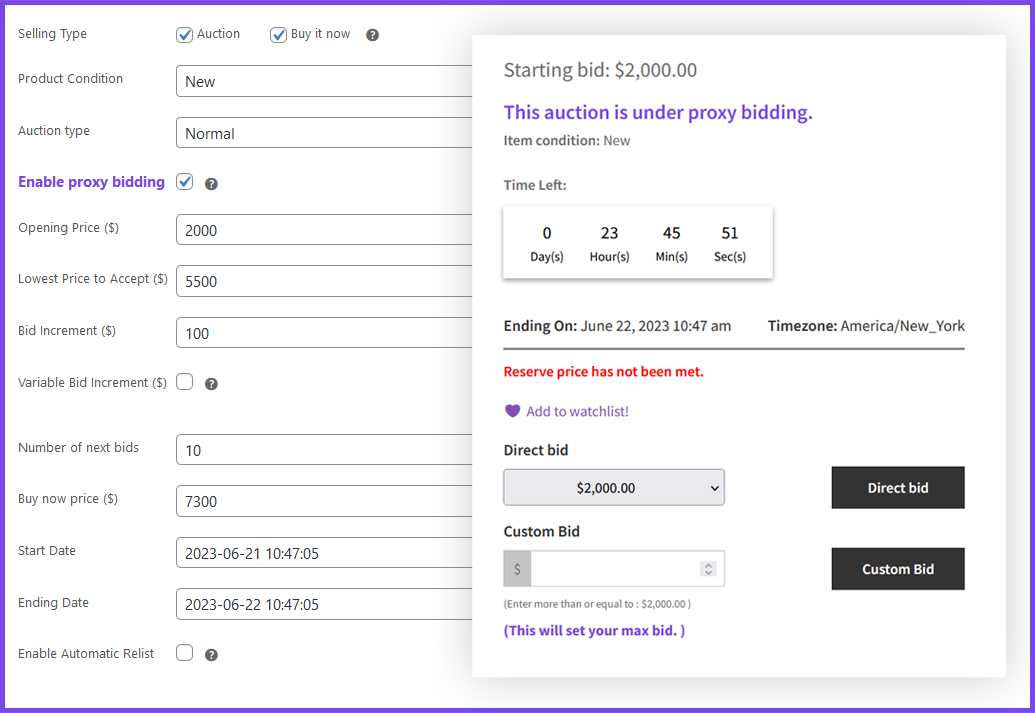Here is your descriptive, detailed caption:

"Screenshot of an online auction listing interface with a distinctive purple trim border. The central section displays two selling types: 'Auction' and 'Buy It Now', both currently selected. Next to these options is a gray question mark for further information. The product condition is specified as 'New'. Under 'Auction Type', the setting is 'Normal'. There is an option for 'Enable Proxy Bidding', highlighted in purple and checked yes, also accompanied by informative question marks. 'Opening Price' is set at $2,000 while the 'Lowest Price to Accept' is stated as $5,500. The 'Bid Increments' are fixed at $100 with 'Variable Bid Increment' yet to be determined. The number of 'Next Bids' is 10. The 'Buy It Now' price is $7,300. The auction's start date is shown as 2023-06-21 at 10:47:05, with the same end time the following day, 2023-06-22 at 10:47:05. 'Automatic Bidding' is enabled with a starting bid of $2,000, and the time remaining is 23 hours and several minutes. Bidders have the option of placing a 'Direct Bid'. The reserve price has not been met. Please note, this information might be outdated as indicated by the current 'Buy It Now' price of $7,300."